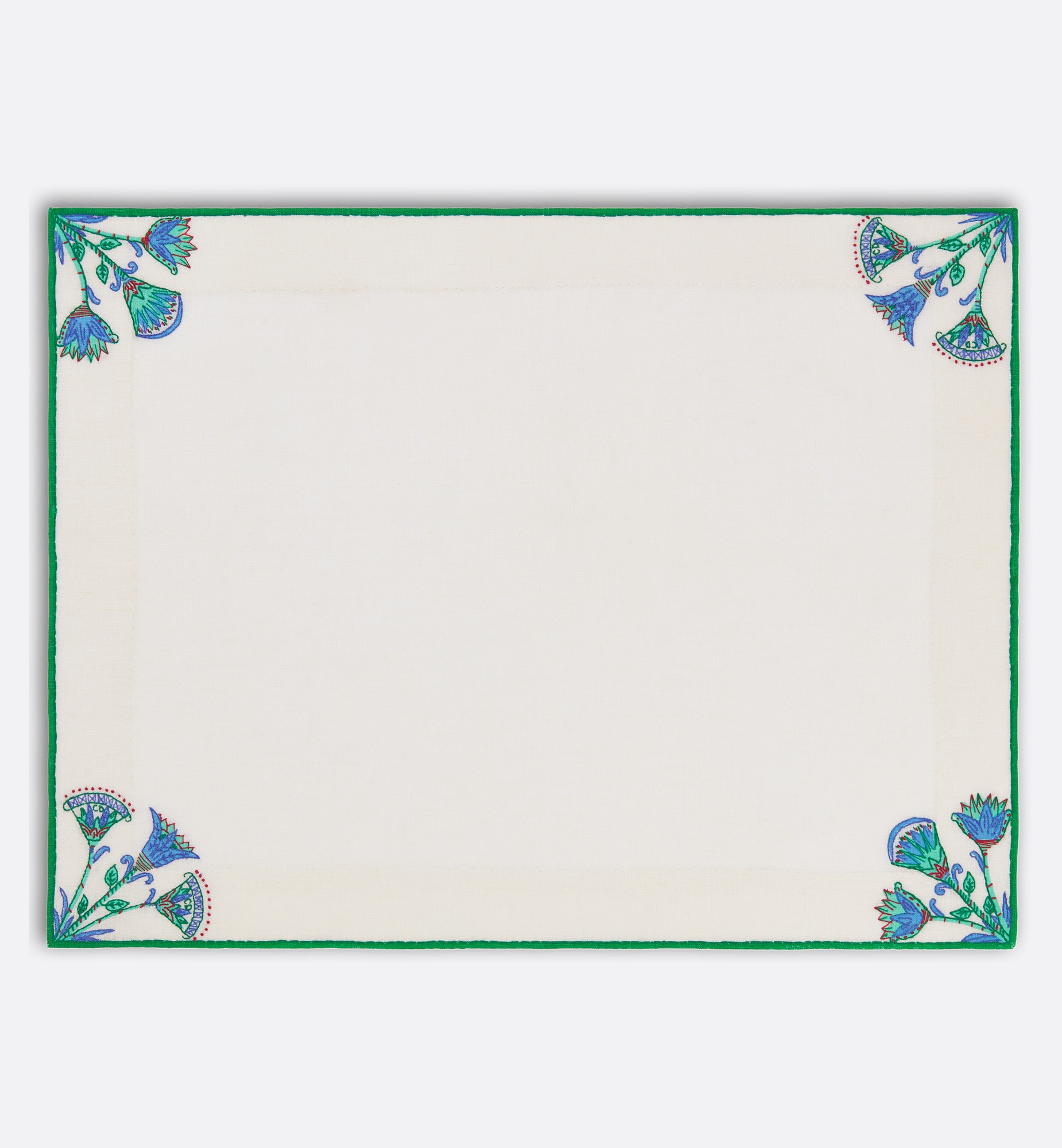The image resembles a decorative piece of paper or an old-fashioned note card with a light gray or cream background that mimics a wall. The central area is a large white rectangle, surrounded by a faintly pink or beige frame that blends subtly with the center. Encircling this is a distinct green border. In each of the four corners of the green border, there are clusters of stylized, hand-drawn flowers. Each cluster consists of three blue and green flowers with red tips, shaped somewhat like 'V's. In the clusters, the flowers are arranged such that the middle flower is slightly larger and either open or closed, contrasting with the surrounding flowers which adopt the opposite state. This pattern repeats across corners: the upper-left and bottom-right corners feature clusters with the middle flower closed, while the upper-right and bottom-left corners have clusters with the middle flower open. The flowers in these corners face towards the opposite diagonal corners. The overall effect is that of a sophisticated, vintage-inspired print with a symmetrical floral motif.